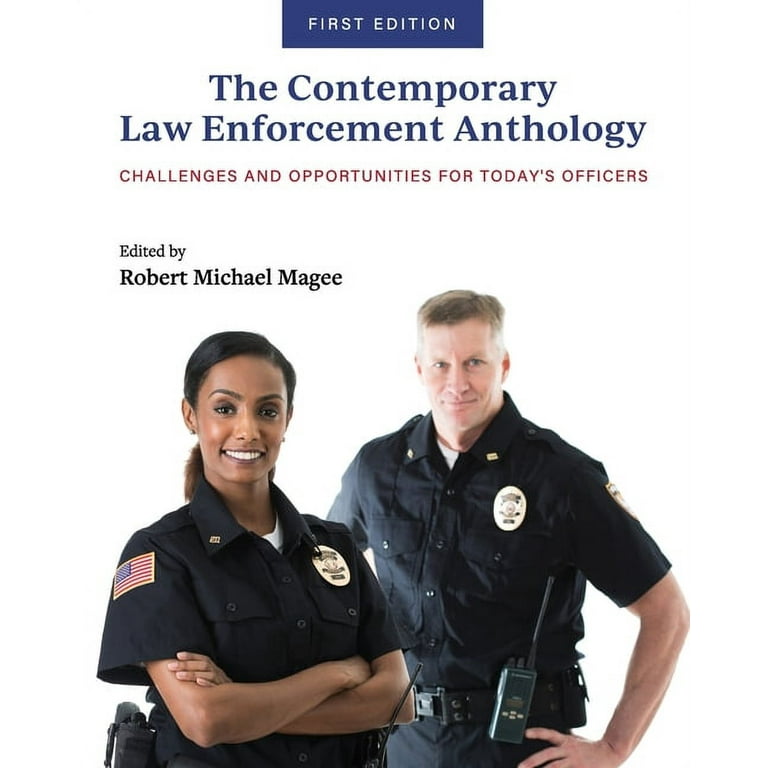The image is a scan of a book cover, which is rectangular in shape with the left and right sides being twice as long as the top and bottom sides. The cover features a solid white background with distinct elements arranged vertically. At the very top, a horizontal blue rectangle contains the text "First Edition" in small white print. Below this, two lines of large blue text read "The Contemporary Law Enforcement Anthology." Further down, in small red print, the subtitle "Challenges and Opportunities for Today's Officers" is displayed. On the left-hand side beneath the subtitle, two rows of small black print state "Edited by Robert Michael Magee."

The lower portion of the cover features a photograph of two police officers from the waist up. The officer on the left is an African-American woman, smiling confidently with her arms crossed. She wears a black, short-sleeved, button-up collared shirt with a large gold-colored badge and an American flag on her sleeve, a pistol in a holster on her right side, and a walkie-talkie on her left. The officer on the right is a Caucasian man with a timid smile, also in a black, short-sleeved, button-up collared shirt with similar badges and gear as his female counterpart. Both officers are looking directly at the camera.